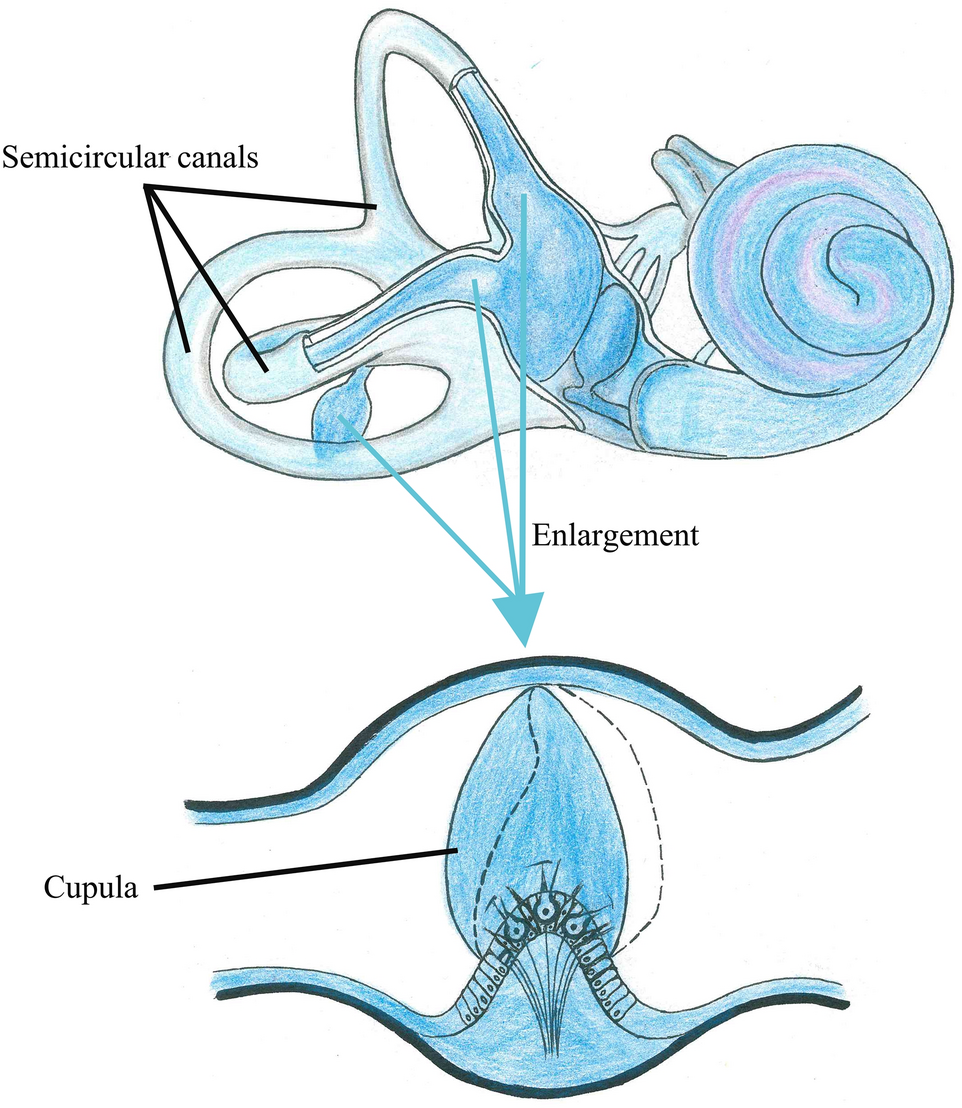The image is a detailed line art illustration of the inner ear, specifically highlighting the semicircular canals and cupula. The upper part of the image is a broad depiction in blue, showing the intricate loops and circles of the semicircular canals with black outlines. This section is labeled "Semicircular Canals." An arrow labeled "Enlargement" points from this area to a close-up view below. This close-up zooms in on a specific part of the semicircular canal, featuring a pear-shaped structure known as the cupula, which sits on a small mound. The cupula is depicted with small hairs in front, indicating its role in maintaining balance. The image is colored neatly within the lines, primarily in blue with a touch of purple around specific areas, giving it depth despite a somewhat cartoony, crayon-filled appearance. The detailed labels and callouts provide a clear understanding of the ear's anatomy, emphasizing the semicircular canals and the cupula's function.